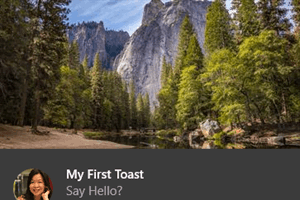The image presents a stunning, albeit subtly surreal, outdoor scene captured in rich color against a stark white background, suggesting it may be AI-generated. The left and right sides of the image are dominated by dense pine forests, their trunks and branches casting intricate shadows on the forest floor, which is a mix of brown dirt and scattered rocks. At the center of the scene, a serene stream meanders through, with the water perfectly mirroring the surrounding rocks and towering pine trees. In the background, majestic cliff-like mountains rise, their rugged, gray faces highlighted with taupes, blacks, and patches of white, topped with hints of light moss. The sky, predominantly visible in the upper left corner, is a brilliant blue with delicate, wispy white clouds drifting across. Beneath this picturesque scene, a gray banner displays a circular image of a woman's face accompanied by the text, "My First Toast. Say hello."